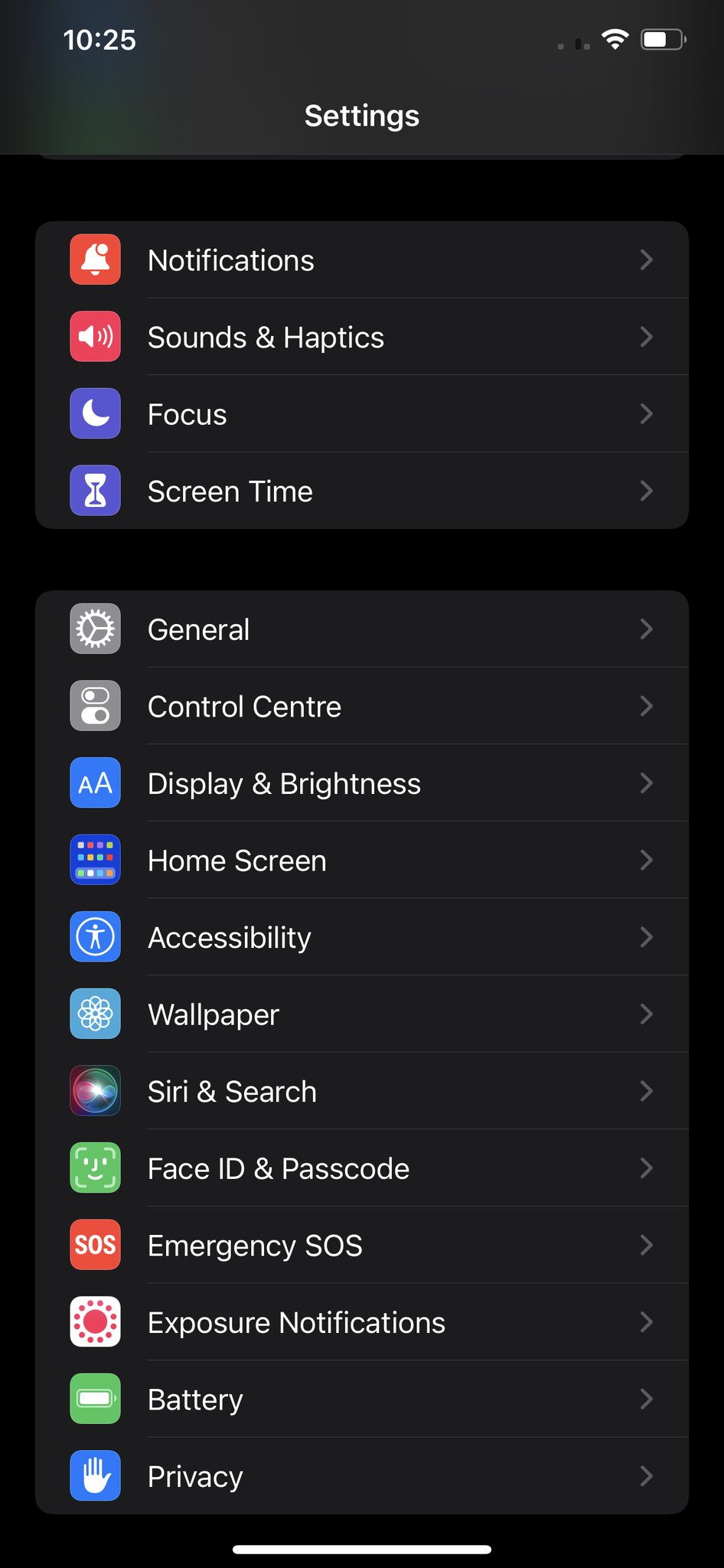The screenshot is from an Android device in dark mode, featuring a black background with white text. At the top-left corner, the time is displayed as 10:25. On the top-right, it shows a symbol labeled as "full Ythong" beside a battery icon at approximately 50% charge.

Below the top bar, there is a red square icon with a white bell, labeled "Notifications." Following it is a lighter red icon with a speaker symbol, labeled "Sound and Haptics." Next, there is a purple icon with a crescent moon, labeled "Focus," and a lighter purple icon with an hourglass, labeled "Screen Time."

Further down, there is a green icon featuring a gear, labeled "General." Below this, there is a toggle switch labeled "Control Centre," styled with the British spelling (Centre). An icon with an uppercase and lowercase "A" in blue is labeled "Display & Brightness."

Continuing the list, options such as "Home Screen," "Accessibility," "Wallpapers," "Siri & Search," "Face ID & Passcode," "Emergency SOS," "Exposure Notifications," "Battery," and "Privacy" are visible. Each of these settings has a grey arrow on the right-hand side, pointing to the right.

The screenshot makes it evident that this is an iOS device due to the presence of Siri and specific feature names.